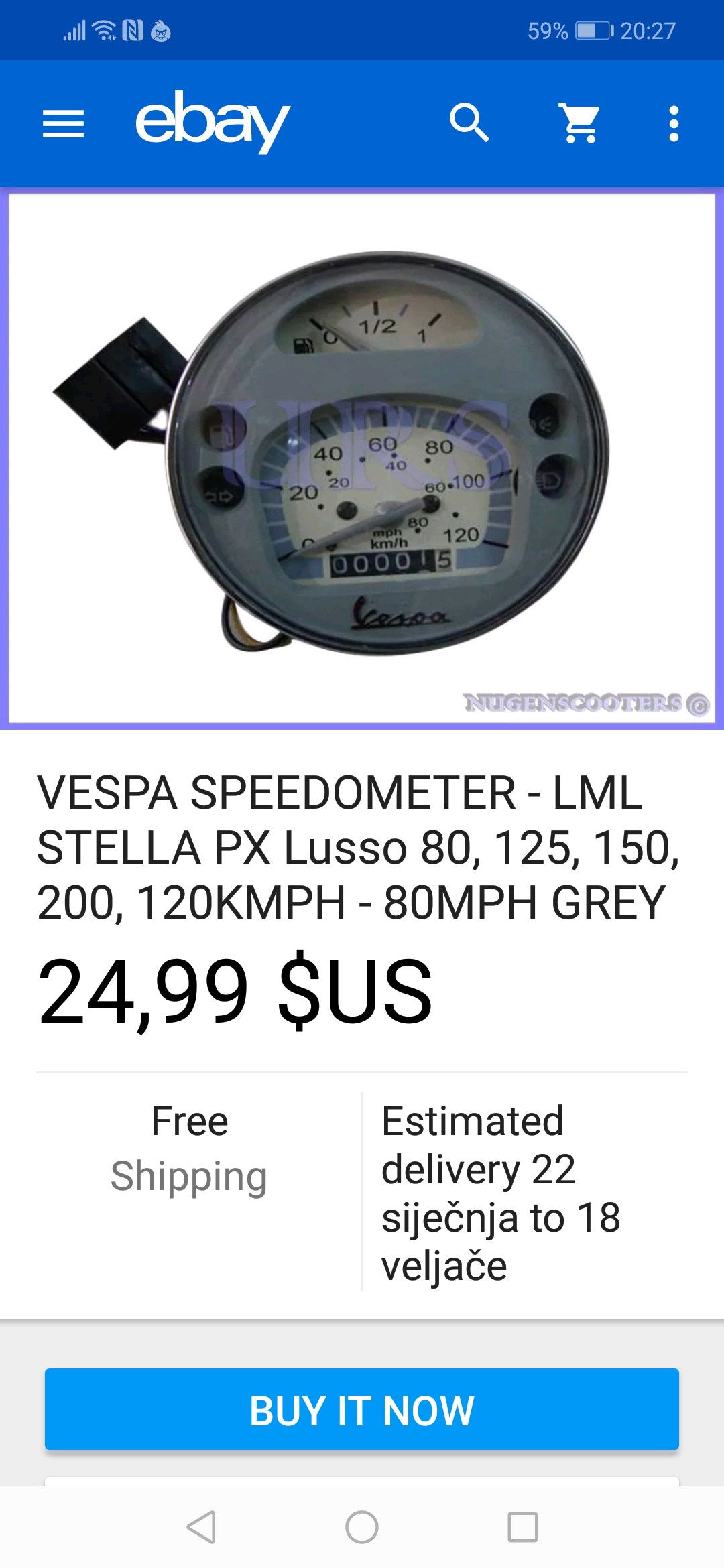The image captures a screenshot taken from a mobile device displaying an eBay listing. The device shows several bars of cellular service and is connected to Wi-Fi. At the top-right corner, alongside the Wi-Fi icon, are two logos likely associated with the phone's network provider. The battery is at 59%, as indicated by the percentage and accompanying icon. The time is 20:27, presented in a 24-hour format.

The eBay interface features a blue banner with white text. On the left, the menu icon (three horizontal lines) provides access to account options. Following that is the eBay logo, then a magnifying glass icon for search, a cart icon, and three vertical dots for additional options.

The listing shown features a photograph of a speedometer. The title reads: "Vespa Speedometer LML Stella PX Lusso 80, 125, 150, 200, 1 to 120 KMPH to 80 MPH Gray". The item is priced at $24.99 USD with free shipping. The estimated delivery date ranges from the 22nd to the 18th of an unspecified month, which is written in a foreign language.